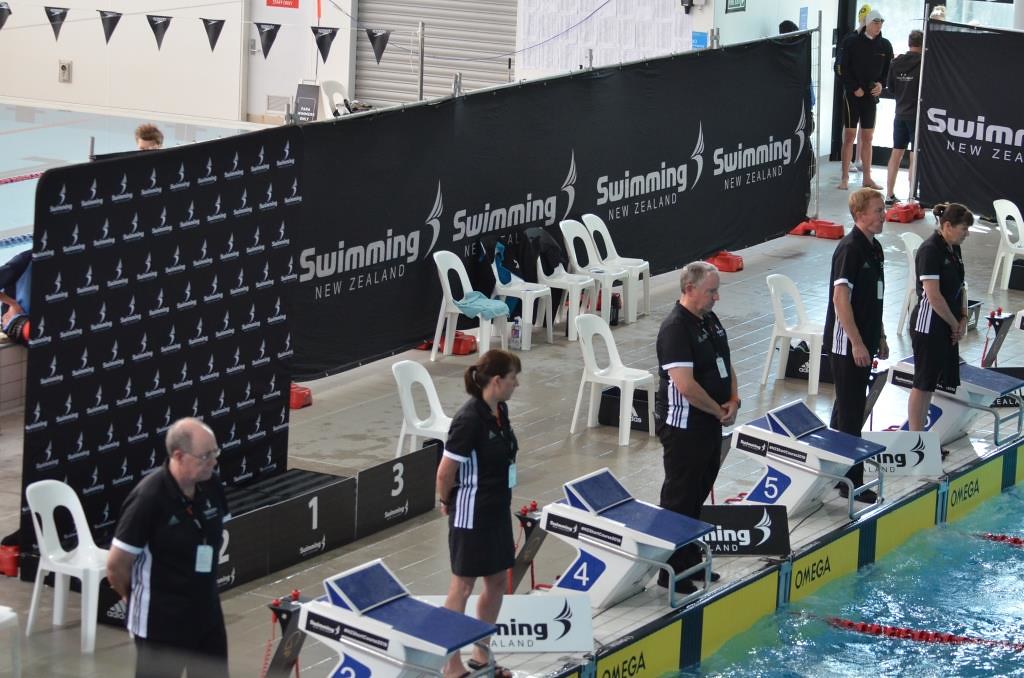This photo, taken at a swim meet in New Zealand, captures a detailed scene at the end of a swimming pool. In the foreground, you can see the corner of the pool with red lane dividers and wet blue starting blocks where swimmers begin their races. Standing next to each lane, observing closely with hands either behind their backs or in front of their waists, are about five officials. They are dressed uniformly in black shirts with white side striping, with the men wearing pants and the women in skirts. Surrounding the area are white chairs scattered with clothing and bags. Dominating the background is a large black banner with "Swimming New Zealand" prominently displayed. Beyond this, the scene extends to another pool on the opposite side of the wall and a doorway where a few swimmers can be seen. Near the left background, there is a podium area for awarding medals to first, second, and third-place victors. The overall atmosphere suggests a highly organized event, with officials ensuring fair play and spectators observing the competition.